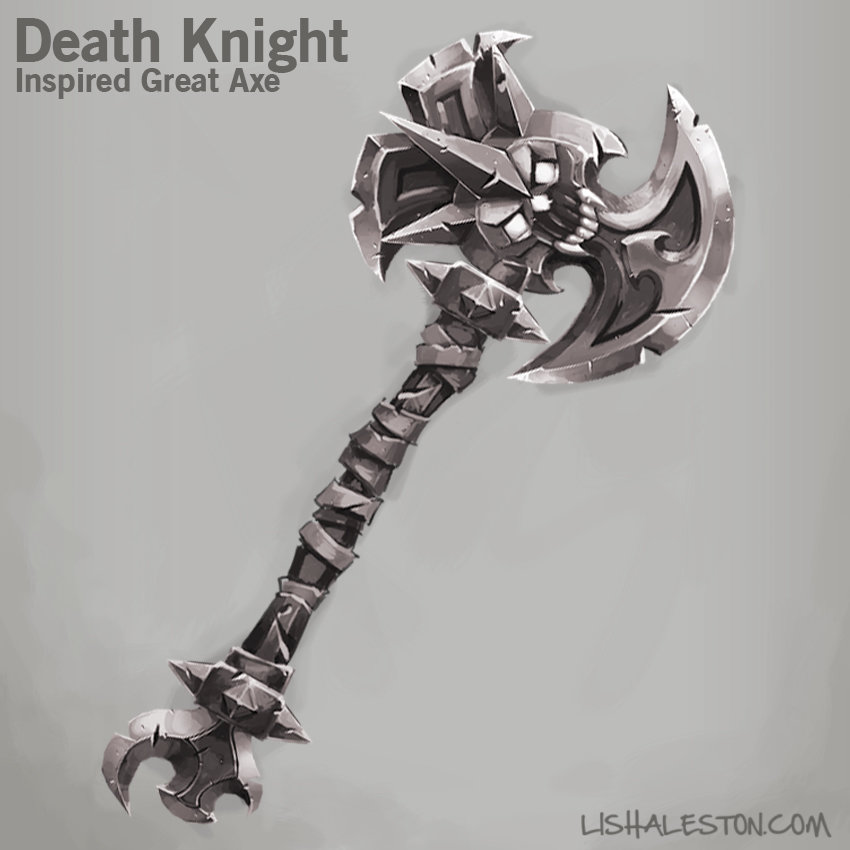This digital art piece showcases a Death Knight Inspired Great Axe, depicted at an angle from the bottom left to the upper right against a stormy, light gray background. The axe, which appears to be a massive, formidable weapon suited for a video game setting, features a metal blade with visible chips and a dark gray handle wrapped with strips of metal. Notably, the head of the axe includes a skull with spikes emanating from it, enhancing its menacing appearance. The handle also appears slightly spiky, adding to the intimidating design of the weapon. In the upper left corner of the image, the text "Death Knight Inspired Great Axe" is prominently displayed, while the lower right corner features the URL "LizHalston.com" in all capital letters, suggesting the artist's website. The detailed and animated nature of the artwork underscores its larger-than-life, video game-inspired aesthetic.